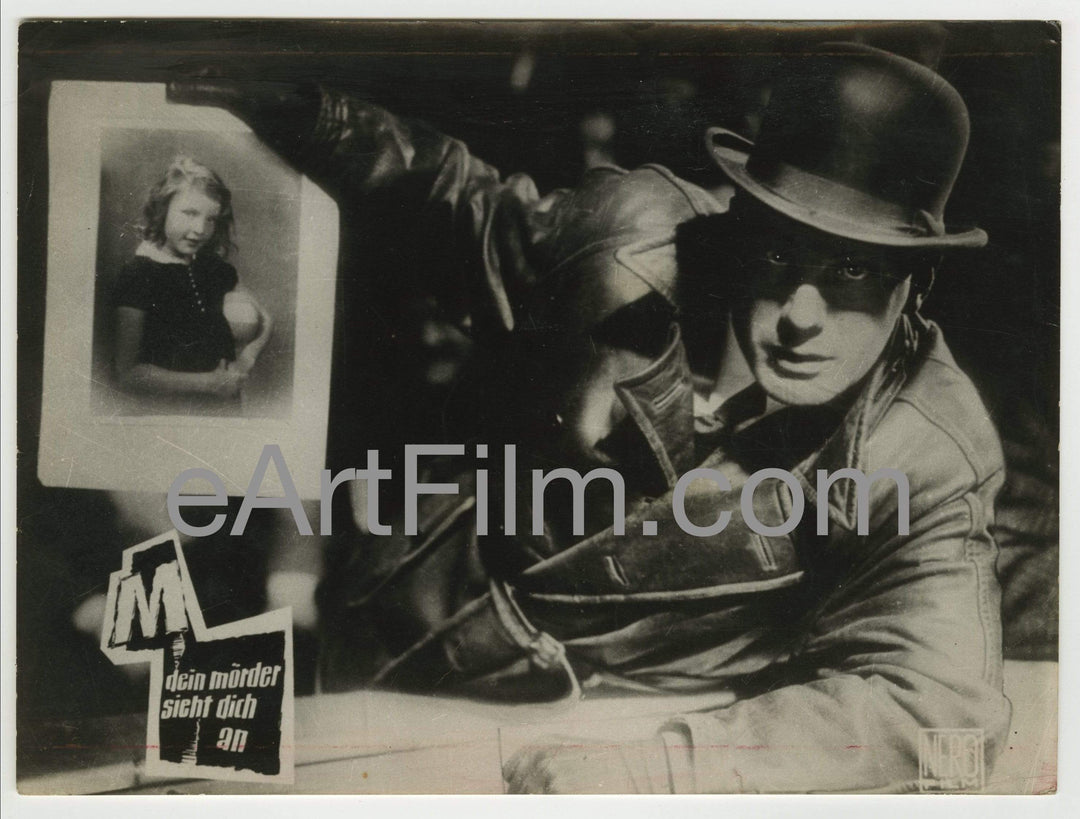A black-and-white photograph captures a somber-looking white man, potentially an old-time movie star, adorned in a black top or derby hat with a black headband. He wears a distinct German-style World War II leather jacket featuring a long collar and black gloves, lending an eerie undertone to the image. The man's expression is serious as he holds up a photograph of a young girl, likely a toddler or early elementary school-aged, with short shoulder-length hair. The girl, dressed in a dark-colored dress with buttons near the top, clutches a small ball under her arm. A watermark, reading "eArtFilm.com" in gray Arial sans serif font, stretches across the middle of the photo, with the letters A and F capitalized. Another logo beneath it reads “M” followed by the phrase “Dissen Mörder Dich Au,” suggesting some German influence. The unsettling aura of the image is heightened by the man's black gloves and the ambiguous context surrounding the photograph of the young girl, evoking a sense of mystery and possible foreboding.